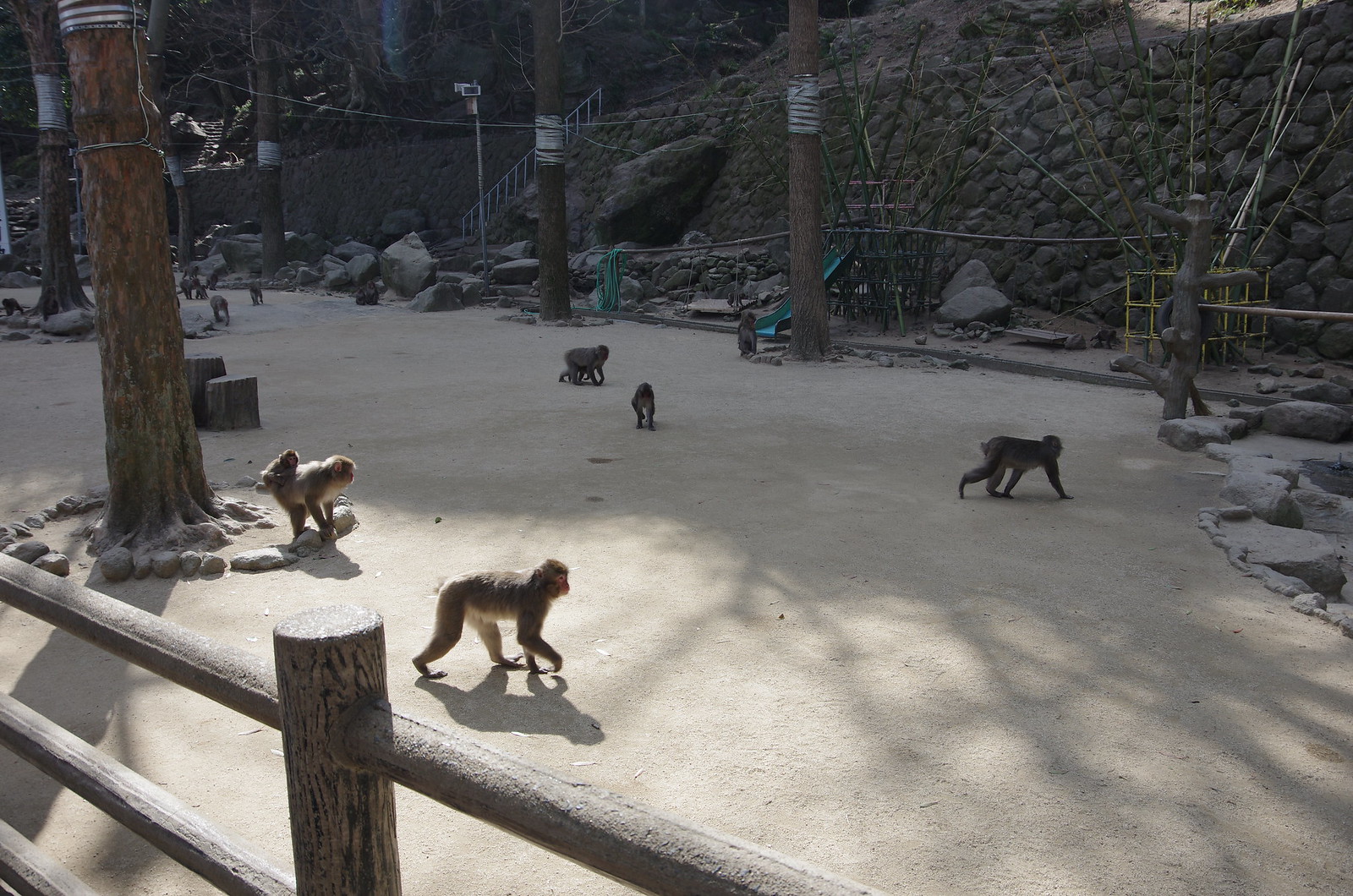This photograph captures the monkey enclosure at a zoo, viewed from an elevated perspective. The top one-third of the image shows the tree line above a large stone wall, approximately 20 feet high, constructed from piled-up rocks. In the enclosure's center stands a massive rock structure that climbs almost to the top of the brick wall, flanked on either side by tall telephone poles. On the right side, two additional large poles are surrounded by rocks at their bases. The ground is a light brown, sandy color, with shadows from nearby trees suggesting the photo might have been taken at dusk. 

Inside the enclosure, there are at least six monkeys, possibly baboons, moving about. One monkey, noticeable for carrying a baby on its back, stands near a pole to the left. Another monkey basks in a sunny patch, walking on all fours with its head to the left and tail to the right. Two more monkeys in the far background are heading in different directions, while a fifth monkey, walking on three legs with one limb raised, is towards the center-right of the image. A small wooden structure resembling a tree with baby branches and surrounded by rocks is also present. The enclosure is secured with a fence in the foreground. Various ropes and strings are attached to the tree trunks, allowing the monkeys to swing between them. The primates are mostly brown and engaged in walking on all fours around their habitat.